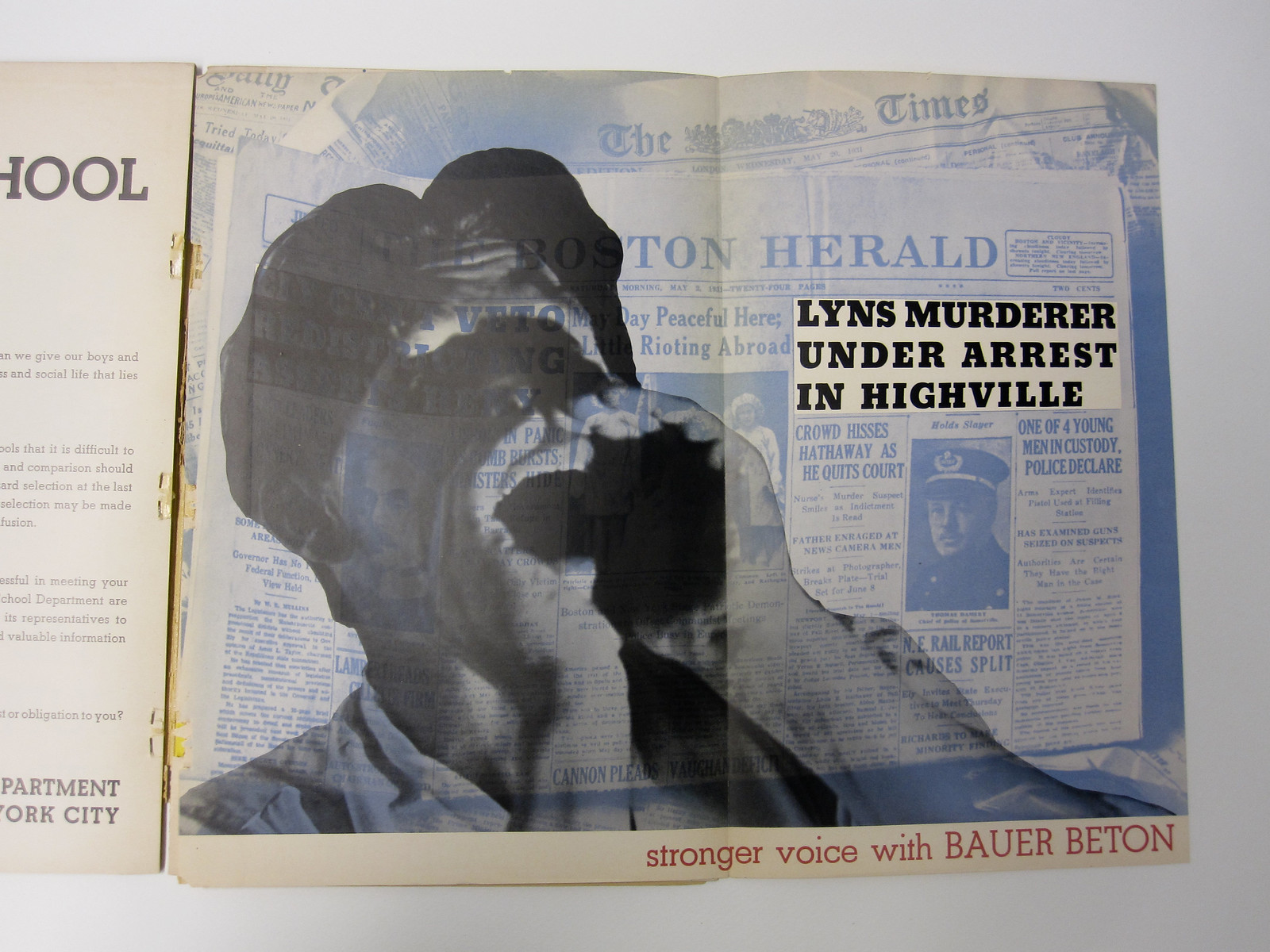The image is a horizontally rectangular composite with a gray outer border, featuring a superimposed black-and-white image of a man overlaid on a blurred background of newspapers. The man, prominently displayed from the upper left to the lower right of the image, has his hands cupped around his mouth as if shouting, with his hair parted in the middle. The newspapers in the background are faint, except for a clear headline in a white banner located on the right side of the image that reads, "Lynn's Murderer Under Arrest in Highville," in black text. Additional text on the newspapers appears blue and indistinct. At the very bottom of the image, there is an orange ring containing the text "Stronger by Royce Bauer Beton" in orange print, suggesting it could be an album cover, further adding to the complex layered aesthetic.